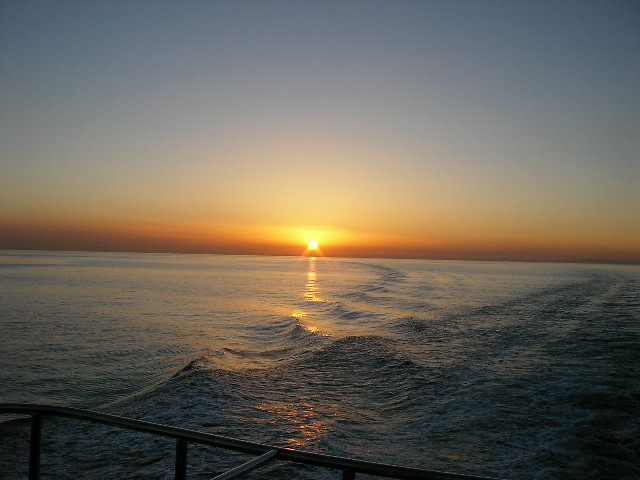This striking image captures the captivating moment of either a sunrise or sunset over a body of water, possibly an ocean, bay, or lake. The sun is positioned just at the horizon, where it meets the water, casting a mix of yellow, orange, and grey hues across the sky and its reflection on the water's surface. The waves below are gently crashing and ripple slightly, their dark grey-blue tones contrasting with the softer sky. The photograph seems to have been taken from a dock or balcony, as indicated by the steel railing visible in the bottom left corner. The horizon holds a darker hue, transitioning from the purple and grey-blue of the sky, suggesting the tranquil yet transient beauty of dawn or dusk. The overall scene conveys a peaceful yet dynamic interplay between light, water, and sky.